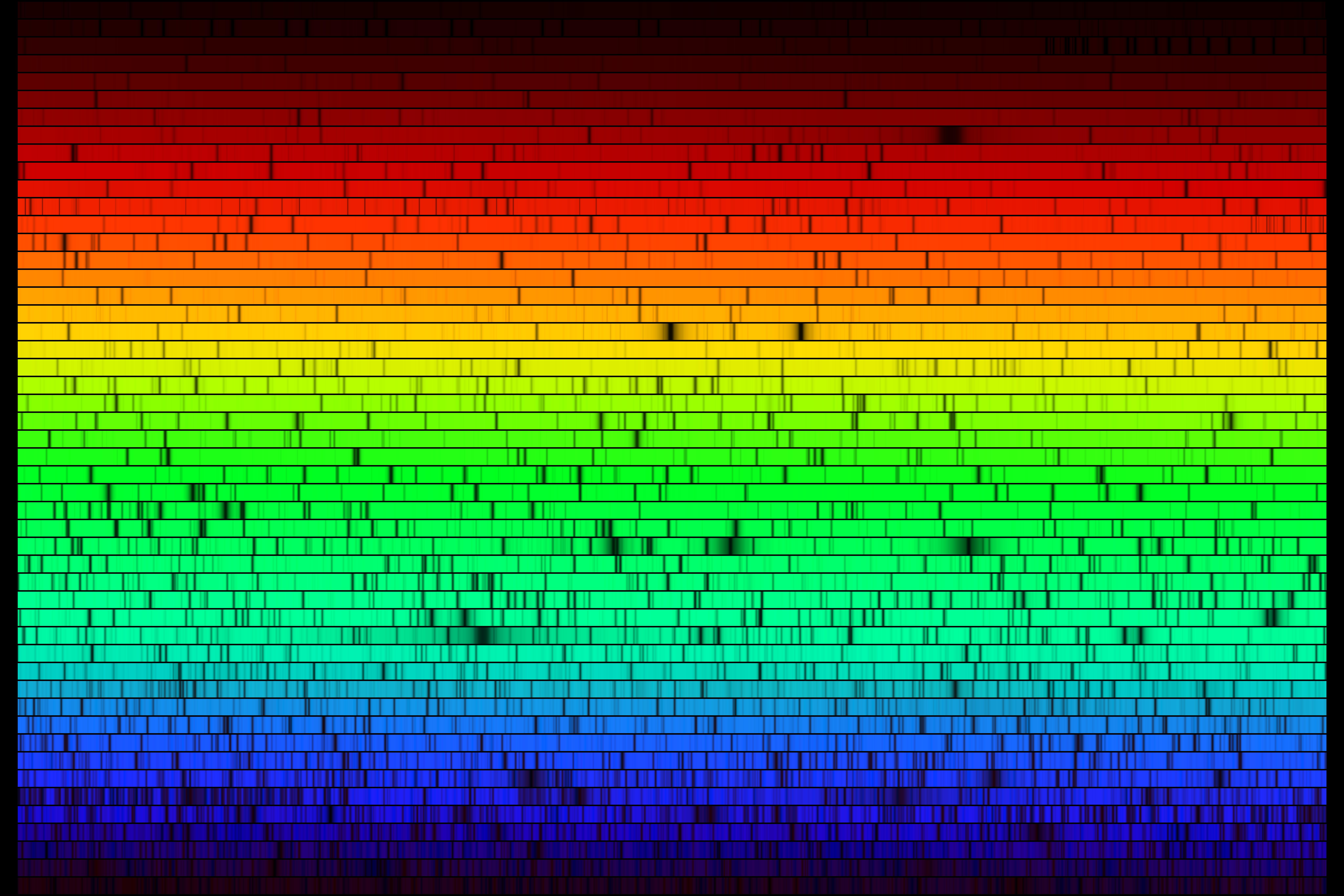The poster is a detailed scientific color chart in a horizontal landscape orientation, featuring a precise depiction of the solar spectrum. It is rectangular with the top and bottom sides twice as long as the left and right sides, framed by a thin black border on all edges. The main area consists of multiple small rectangles and squares arranged like a brick wall, each filled with vibrant colors that blend into each other to create a smooth gradient effect.

At the very top, the colors start with pitch-black, transitioning into dark red, then a vibrant red, followed by orange and yellow. The center is dominated by a bright green, which gradually fades into greenish-blue, then into dark blue and purple, and finally back to black at the bottom. 

Overlaid across the entire poster are numerous horizontal black lines intersected by short vertical segments that vary in placement and density. These lines become more frequent and closer together towards the lower part of the poster, while they are more spaced out and less frequent towards the top. The intricate pattern of these lines creates a complex, textured appearance, adding to the poster's detailed and high-resolution representation of the solar spectrum.